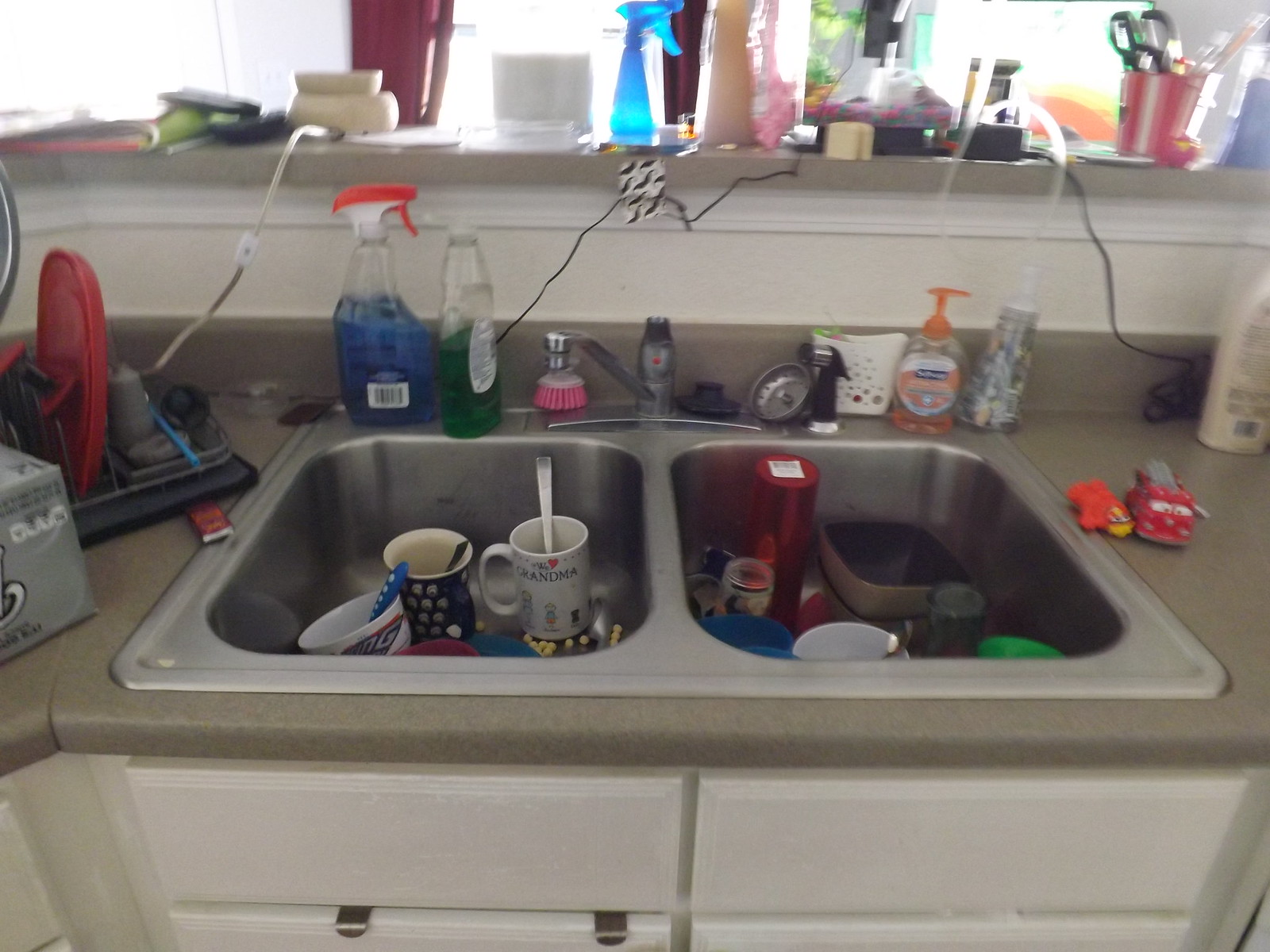This photograph captures a cluttered, silver double sink filled with various items. Inside the sink, there are several coffee mugs containing spoons, along with a few discarded plastic water bottles. To the left of the sink on the counter, there is a spray bottle filled with blue liquid, a clear bottle containing green liquid, and a pink dishwashing brush. A soap dispenser is also present. Below the sink, white cabinet doors are visible. 

The counter itself has a brown, marble-like appearance. To the left of the counter, a draining board and a case of soda are positioned. On the right side, two small toys rest on the counter, and black cords run upwards. Above the sink, an overhead cabinet is cluttered with various indistinguishable items, including another blue spray bottle, though the details are blurred and unclear.